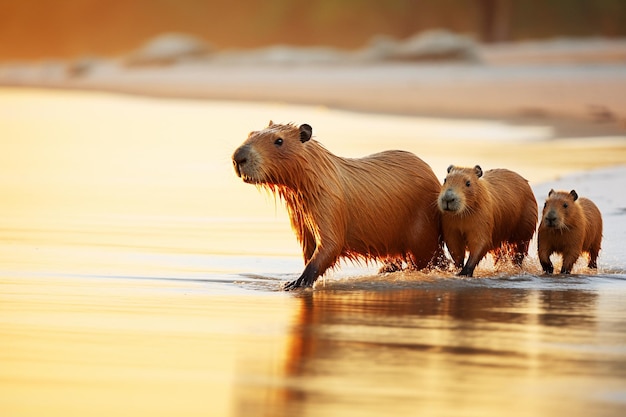A heartwarming image captures a family of sea otters at the shoreline during sunset. The family consists of a mother and her two pups, one significantly larger than the other. The otters have rust-colored fur, accented by black noses surrounded by light tan or white markings. Their delicate whiskers, small ears, and expressive brown eyes add to their adorable appearance. The trio walks on all fours at the water's edge, where gentle waves meet the sand, casting a serene and intimate scene against the backdrop of the setting sun.